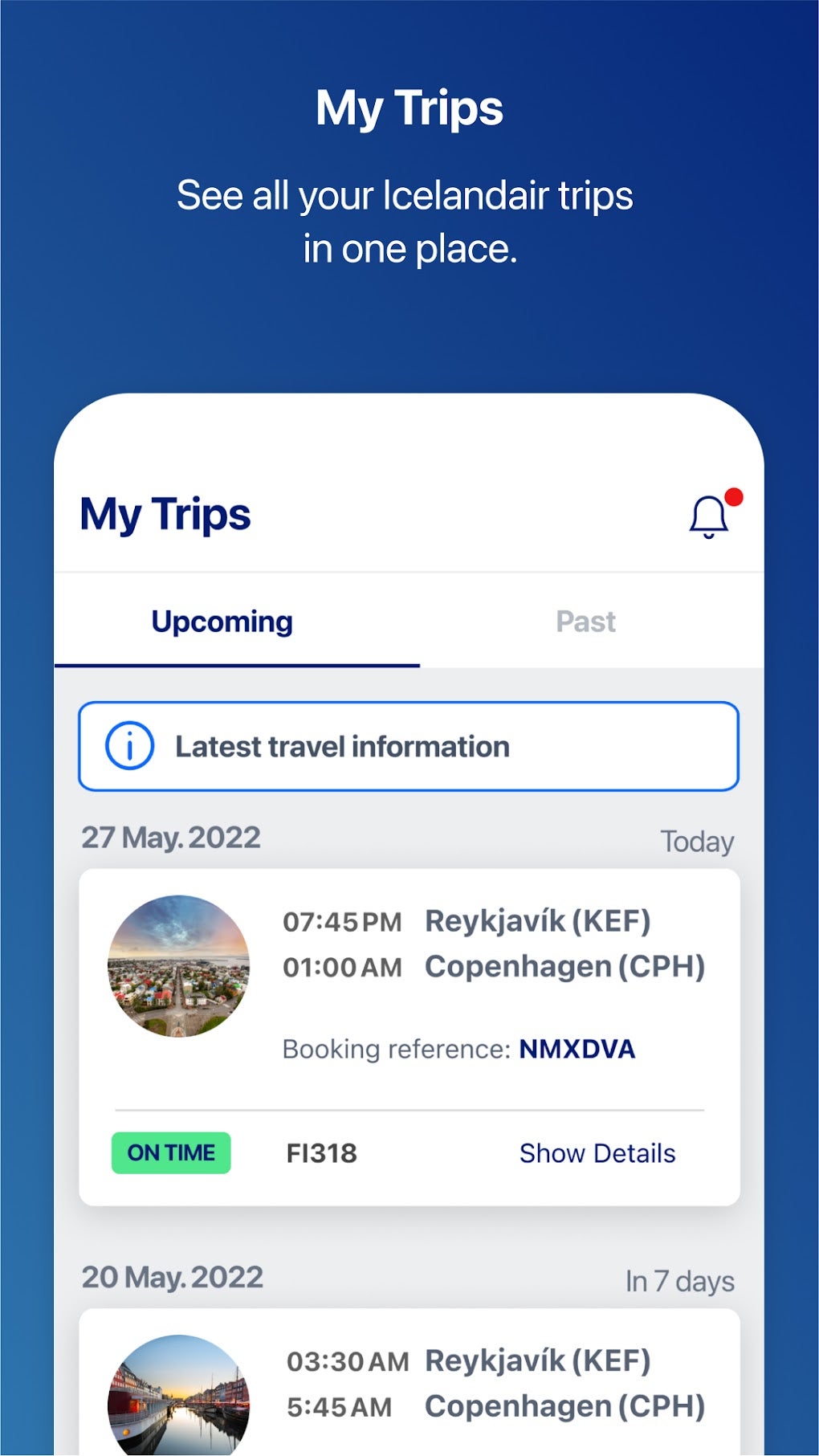Screenshot of the MyTrips website, showcasing all Icelandair trips in one place. The background is a dark blue, complementing the central white background of a phone outline situated in the middle. At the top left of this section, you see the heading "MyTrips." On the far right of the same row, there's an alarm bell icon with a red notification circle next to it.

Below the "MyTrips" heading are two tabs: "Upcoming" and "Past." The "Upcoming" tab is underlined, indicating that it is the current selection. Directly below is a line of text stating "Latest Travel Information" with an information icon beside it, encased in a box with a blue outline. 

A white box below this section features detailed trip information. To the left, outside the box, is the date "27 May 2022." Inside the box, there's an avatar depicting a city skyline accompanied by the text "745 PM Reykjavik" and "1 AM Copenhagen." The booking preference is listed as "NMXDVA," and there's an "On Time" tag in green. The flight number "FI318" is displayed along with a "Show Details" section.

Below this white box is another one with similar trip details. To the left, outside this second box, is the date "20 May 2022." Inside the box, the times are noted as "3:30 AM Reykjavik" and "5:45 AM Copenhagen."